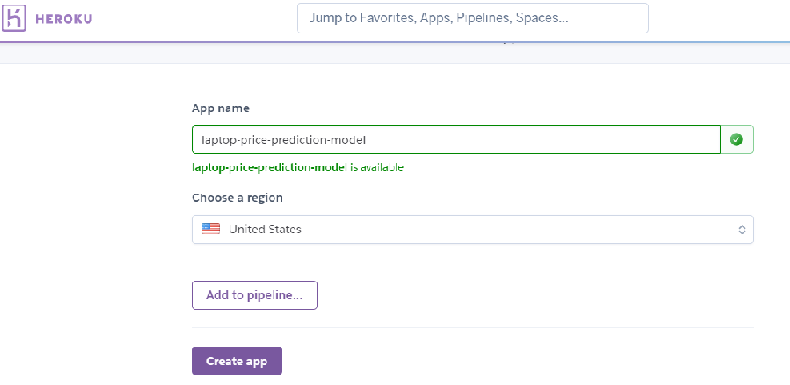The image showcases a webpage from the website Heroku. The word "Heroku" is prominently displayed in purple lettering at the top left corner. Next to this, a purple box contains a stylized purple letter "K". In the center of the page, a long pop-up box appears with the text "Jump to favorite apps", though the wording in the box is slightly unclear.

Below this, the main body of the webpage is visible. It lists an app named "Laptop Price Prediction Model" with some green text written below it, which is not in English. Underneath, there is a section labeled "Choose a region" with "United States" already selected. An image of the United States flag, colored red, white, and blue, is displayed next to it.

Further down, two interactive buttons are present. One says "Add to Pipeline" in purple, enclosed within a purple-outlined box. The other button is labeled "Create App" in white text within a solid purple box. The page appears uncluttered and straightforward, though it does not provide additional context about its specific purpose or which stage of the app development process it pertains to.